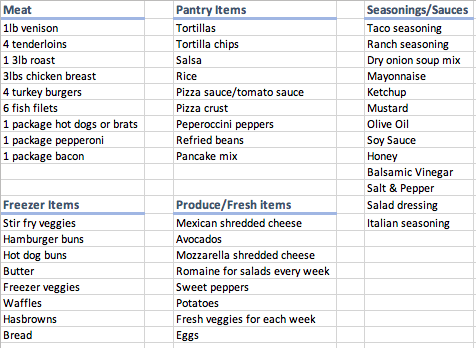Here’s a detailed and cleaned-up caption:

"A detailed screenshot of a shopping list app, presented on a background designed to resemble a lined notebook paper. The list is organized into several categories. The 'Meat' section includes: 1 pound of venison, 4 tenderloins, a 3-pound roast, 3 pounds of chicken breast, 4 turkey burgers, 6 fish fillets, 1 package of hot dogs or brats, 1 package of pepperoni, and 1 package of bacon. Under 'Pantry Items', the list features: tortillas, tortilla chips, salsa, rice, pizza sauce/tomato sauce, pizza crust, pepperoncini peppers, refried beans, pancake mix, seasonings/sauces (including taco seasoning, ranch seasoning, dry onion soup mix), mayonnaise, ketchup, mustard, olive oil, soy sauce, honey, balsamic vinegar, salt and pepper, salad dressing, and Italian seasoning. The 'Freezer Items' category lists: stir-fry veggies, hamburger buns, hot dog buns, butter, freezer veggies, waffles, hash browns, and bread. The 'Produce/Fresh Items' section includes: Mexican shredded cheese, avocados, mozzarella shredded cheese, romaine for salads (weekly), sweet peppers, potatoes, fresh veggies for each week, and eggs."